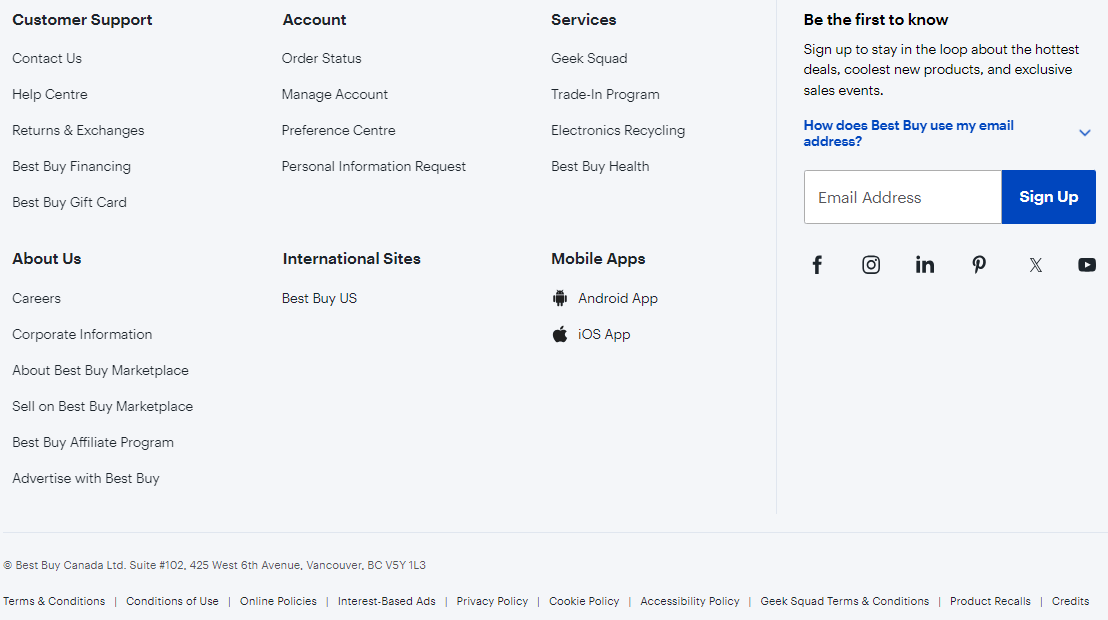This detailed image captures the footer section of a Best Buy website, primarily focusing on customer support and additional services. On the left-hand side, the "Customer Support" header, bolded in black, features prominently. Below it are links for "Contact Us," "Help Center," "Returns & Exchanges," "Best Buy Financing," and "Best Buy Gift Card."

Directly parallel is the "Account" section, prominently listing "Order Status" and, below it, options to "Manage Account," "Preference Center," and "Personal Information Request."

Adjacent to this is the "Services" category, including "Geek Squad," "Trade-In Program," "Electronics Recycling," and "Best Buy Health." 

To the left of this, the "About Us" section details options such as "Careers," "Corporate Information," "About Best Buy Marketplace," "Sell on Best Buy Marketplace," "Best Buy Affiliate Program," and "Advertise with Best Buy."

Nearby, the "International Sites" section lists "Best Buy U.S." Further right, "Mobile Apps" includes the options for downloading the app on Android and iOS, accompanied by their respective icons.

On the far right, separated by a thin line, is a call-to-action section titled "Be the First to Know," bolded in black. Below this heading is a paragraph of body text, followed by the question link, "How does Best Buy use my email address?" highlighted in blue. Directly underneath, there's a field to enter an email address, accompanied by a blue sign-up button. Social media icons are displayed at the bottom.